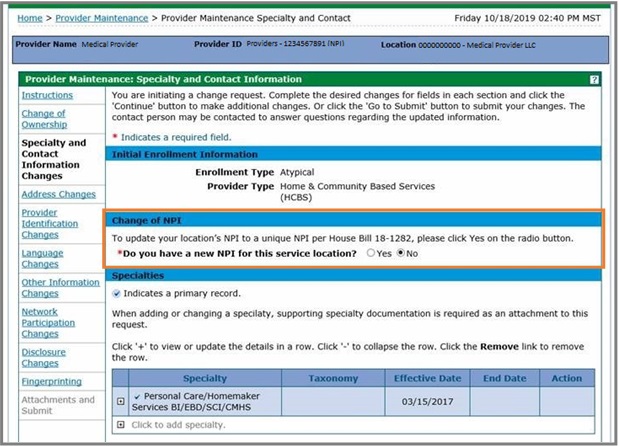The image is a detailed screenshot of an application interface, prominently featuring several sections related to provider maintenance. At the top of the image, there is a blue button labeled "Home". To the right of this button, there are sequentially listed tabs: "Provider Maintenance" in blue, accompanied by an arrow, followed by "Provider Maintenance Specialty and Contact".

The screenshot captures the date and time as "Friday, October 18, 2019, at 2:40 p.m. Mountain Standard Time". Below this timestamp, there's a blue banner displaying key provider details: "Provider Name", "Medical Provider", "Provider ID", showing "NPI", and "Provider Location" with numerous zeros, indicating placeholder information, and "Medical Provider LLC".

Further down, a green banner highlights "Provider Maintenance Specialty and Contact Information". A message within this section indicates that a change request is being initiated. The instructions read: "Complete the desired changes for fields in each section and click the 'Continue' button to make additional changes, or click the 'Go to Submit' button to submit your changes. The contact person will be contacted to answer questions regarding the updated information".

Near the bottom of the image, a blue bar displays "Initial Enrollment Information". It provides specific enrollment details, stating: "Enrollment is atypical", "Provider Type is Home and Community-Based Services", and mentioning a "Change of NPI".